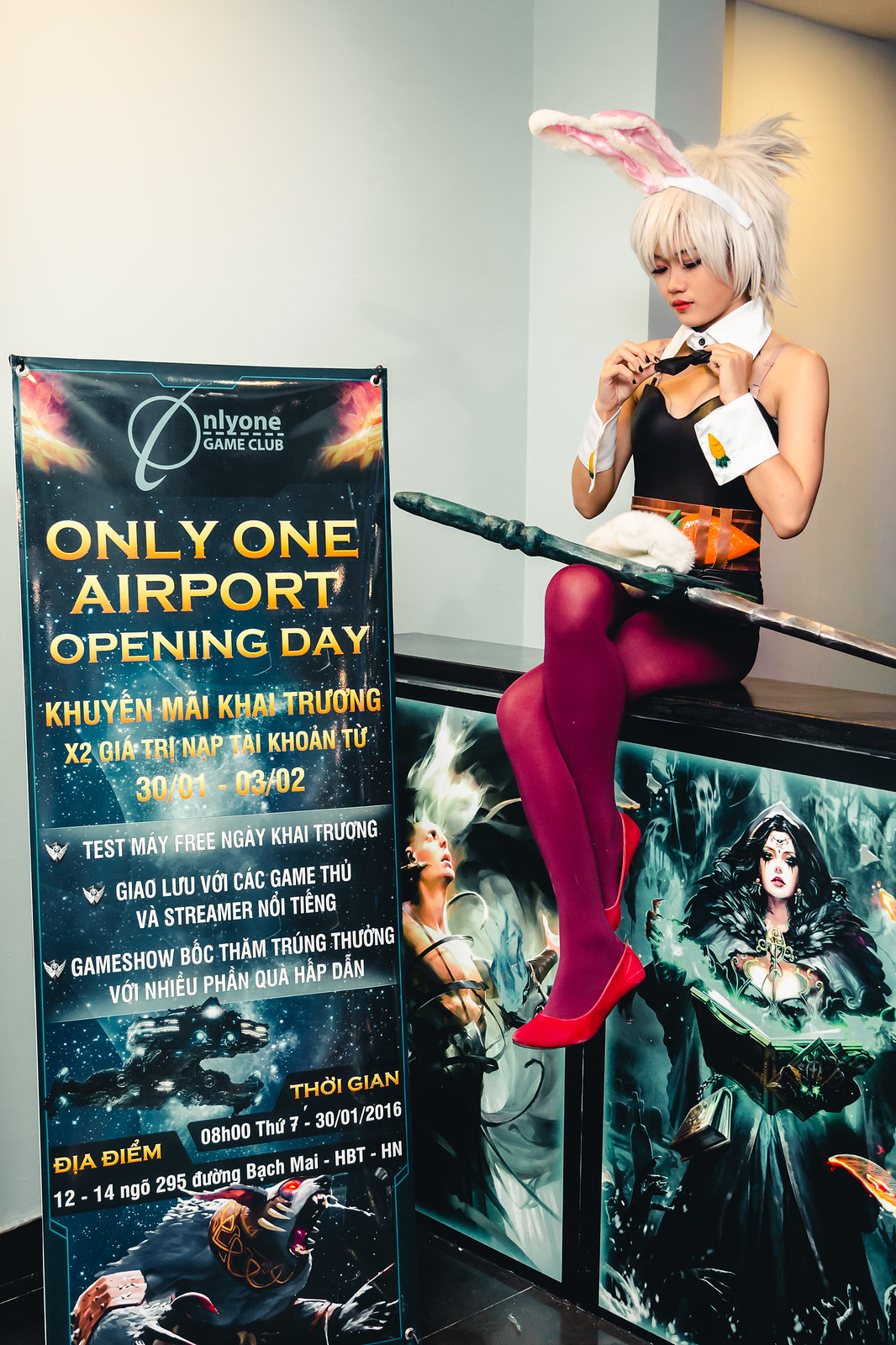A young woman with fair skin, dressed in a black suit paired with red shoes and purple stockings, sits atop an advertisement. Her attire features a white scarf around her neck, white cards adorning her wrists, and a black tie held between her hands. She sports an anime-style appearance with white and pink hair, black eyebrows and lashes, red lipstick, and bunny ears atop her head. Her eyes are closed, and she has a sword resting across her lap over a white cloth. The scene includes an advertisement to the left, displaying the text: "Only One Game Club, Only One Airport Opening Today," followed by a mixture of foreign language and specific details like "30-01-2016" and "Test May Free, Nguy Hi, Turing." The poster backdrop is predominantly black with stars and flames, featuring a gray creature with red eyes and claws. Below the girl, two pictures can be seen: one of a character with dark black hair in a green dress and another of a man with his head tilted back, arms crossed, and a white flame emerging from his face. The setting suggests a possible Vietnamese or Asian origin, with the atmosphere tinted in hues of green, pink, and white.